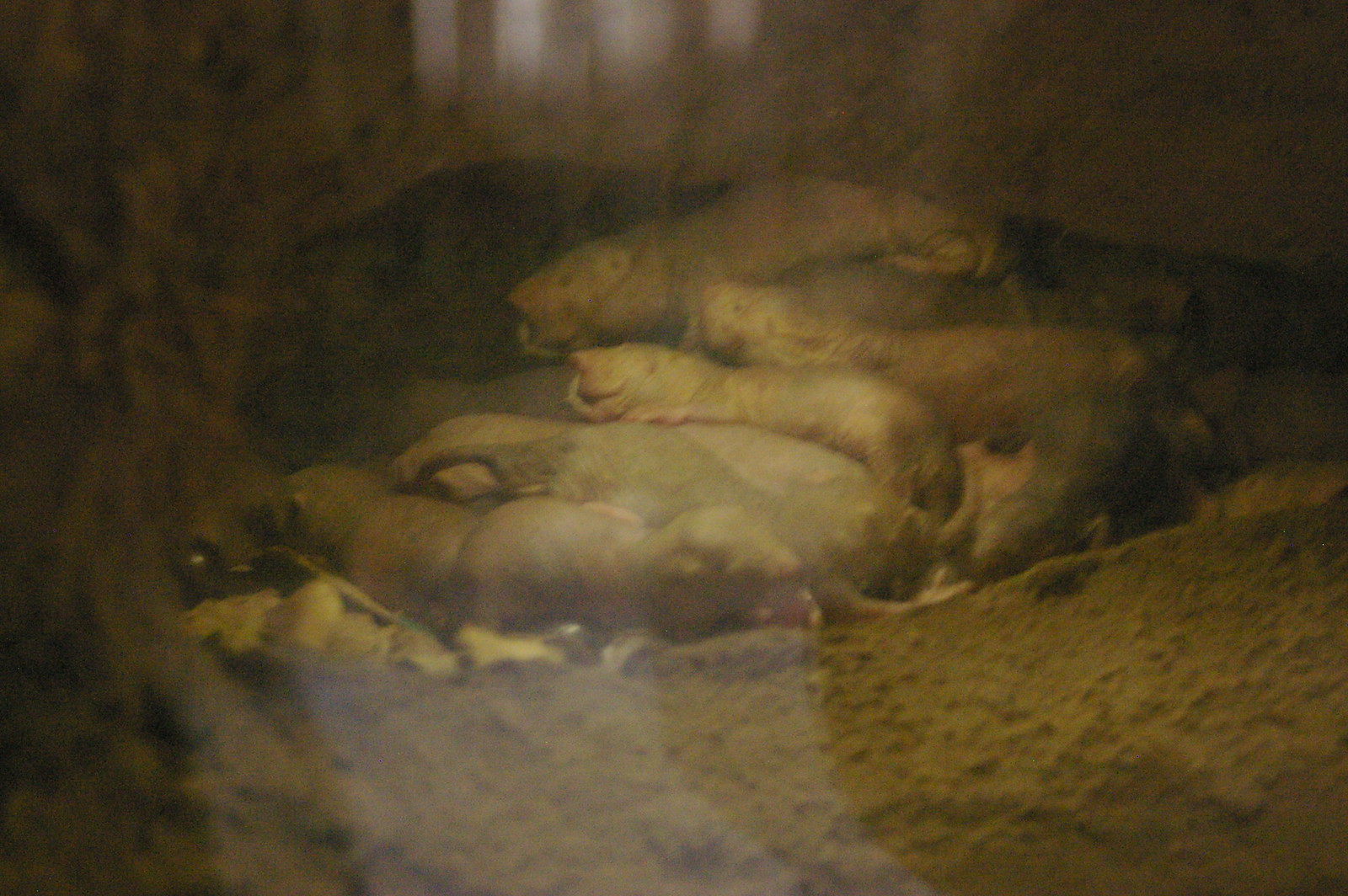The image depicts a dark, cavernous environment with a sandy, beige-hued ground. In this muddy cave-like setting, there are six or seven small animals huddled together, likely for warmth and safety. They appear to be newborns, displaying light gray to white fur. Their long tails suggest they could be rats, gophers, or perhaps even possums. These babies are gathered closely around a larger dark gray animal, presumably their mother, lying on her side as they feed. A single ray of light illuminates this intimate scene within the otherwise shaded and cozy burrow, indicating a well-established and secure dwelling for the animals.